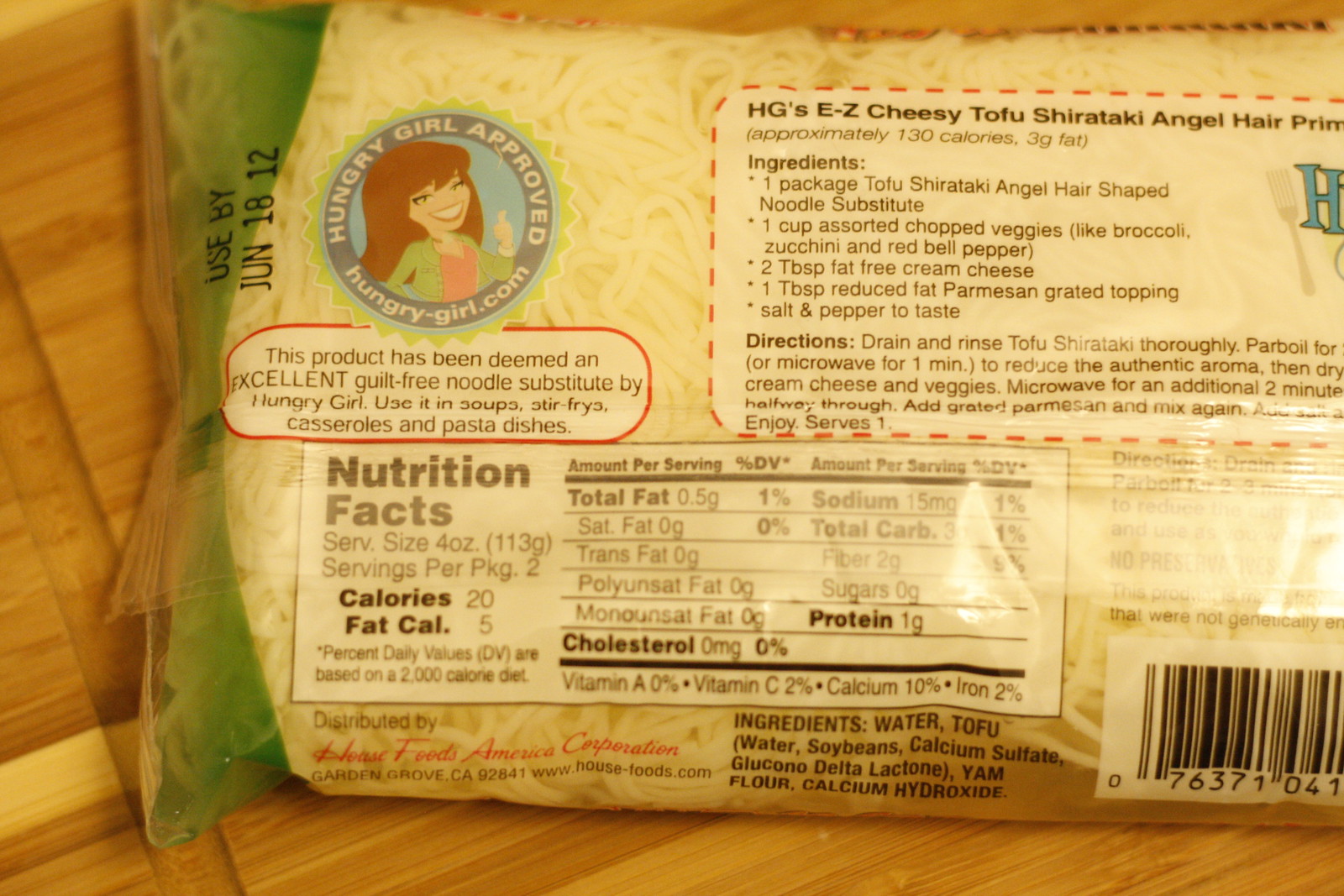The image showcases a package of tofu-based shirataki angel hair noodles, designed as a guilt-free noodle alternative. The noodles, made with a tofu base, bear a similar color to rice but feature a noodle-like texture. Prominent on the package is an expiration date of June 18, 2012. The back label includes a "Hungry Girl Approved" stamp, indicating that the product is endorsed as an excellent guilt-free noodle substitute by Hungry Girl. This endorsement suggests using the noodles in soups, stir-fries, casseroles, and pasta dishes.

The package also features a nutrition facts label detailing the nutritional content and a recipe for "Cheesy Tofu Shirataki Angel Hair Primavera" positioned above the nutrition label. Additionally, there is a barcode for scanning. The product is distributed by House Foods America Corporation, based in Garden Grove, California. The package rests on what appears to be a wooden table or cutting board, identifiable by its texture and a characteristic dip typically found in cutting boards.